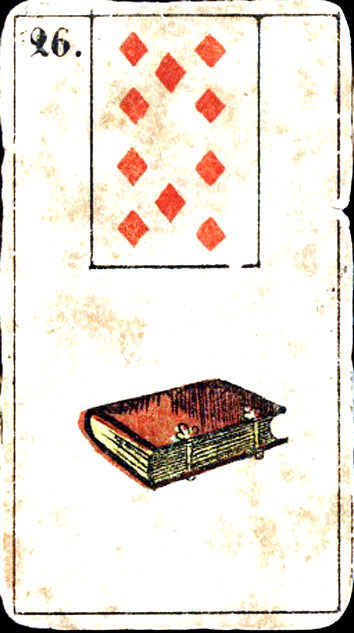The image presents a detailed illustration resembling vintage artwork, centered around two primary elements: a card and a book. The card, appearing aged with frayed edges, is predominantly white and features the number '26' written in the upper left corner. Within the main card, there is a smaller card depicted, adorned with nine red diamonds. Alongside the card, the illustration also includes a thick book encased in a brown binder cover. The book's pages, seemingly gold-leafed, shimmer subtly and are secured by two ornate, gold clasps. This fusion of elements gives the image a historical and antique aesthetic.